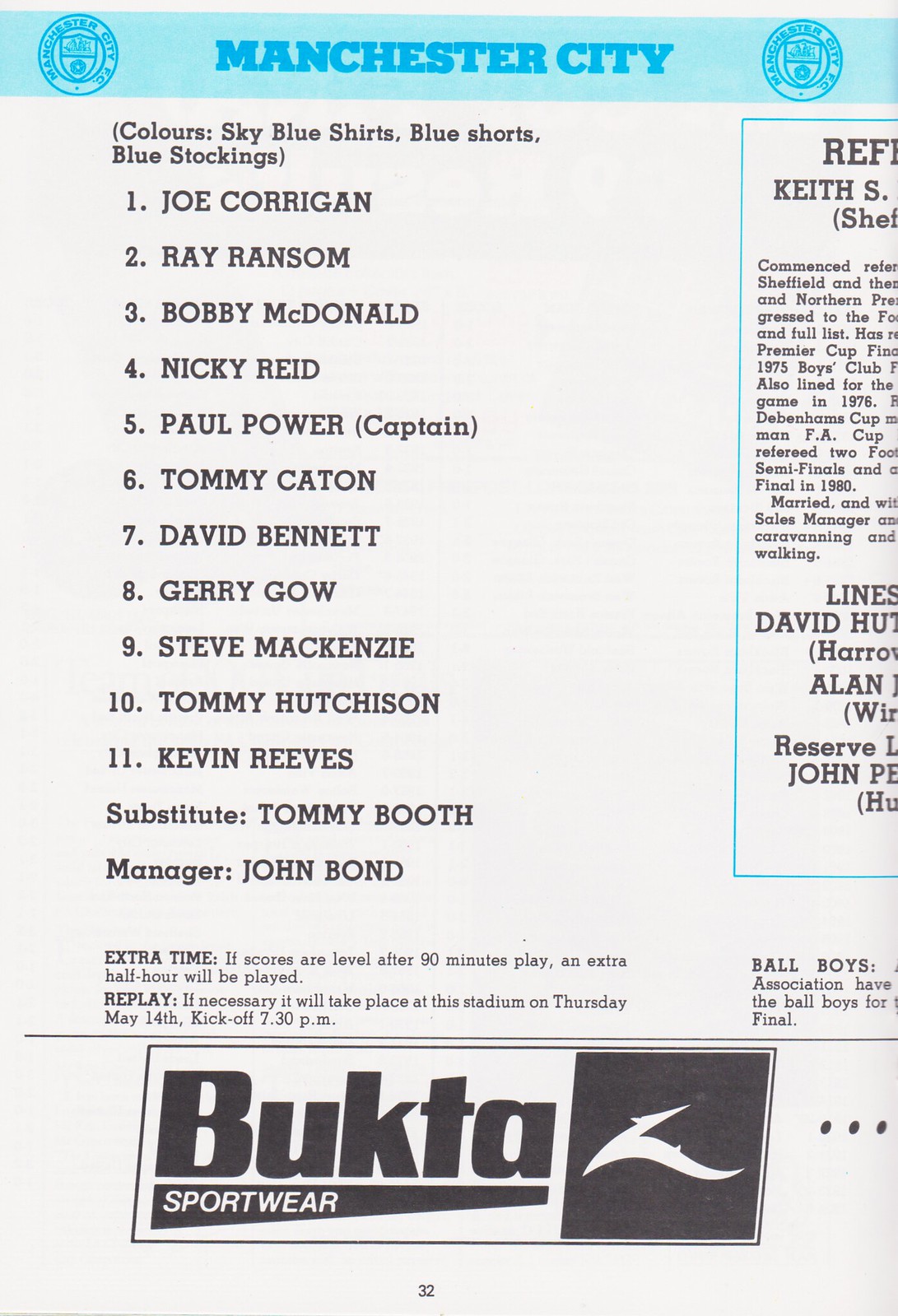This image depicts a program for a Manchester City football team. The top of the program features a light blue horizontal bar with the Manchester City crest in dark blue located on both the left and right corners, and "Manchester City" printed in bold capital letters in the center. Below this header, the program lists the team's colors as "sky blue shirts, blue shorts, blue stockings." 

The players are listed in black capital letters as follows:
1. Joe Corrigan
2. Ray Ransom
3. Bobby McDonald 
4. Nicky Reid
5. Paul Power (Captain)
6. Tommy Caton
7. David Bennett
8. Gerry Gow
9. Steve Mackenzie
10. Tommy Hutchison
11. Kevin Reeves

Following the list of players, the program notes the substitute as Tommy Booth and the manager as John Bond. Beneath the player list, a small, unreadable paragraph of typed text appears to discuss rules concerning extra time and replays.

At the very bottom of the program, a horizontal black line separates the main content from a horizontal advertisement. This ad, which is slanted slightly to the right, features a white background with black lettering spelling "Bukta," underlined by a black swash with the text "Sportswear" in white. The rightmost section of the ad has a black background with a white logo of a bird in flight. The right edge of the image shows the cut-off portion of another article, which includes a headline and a body of text that are too small to read.